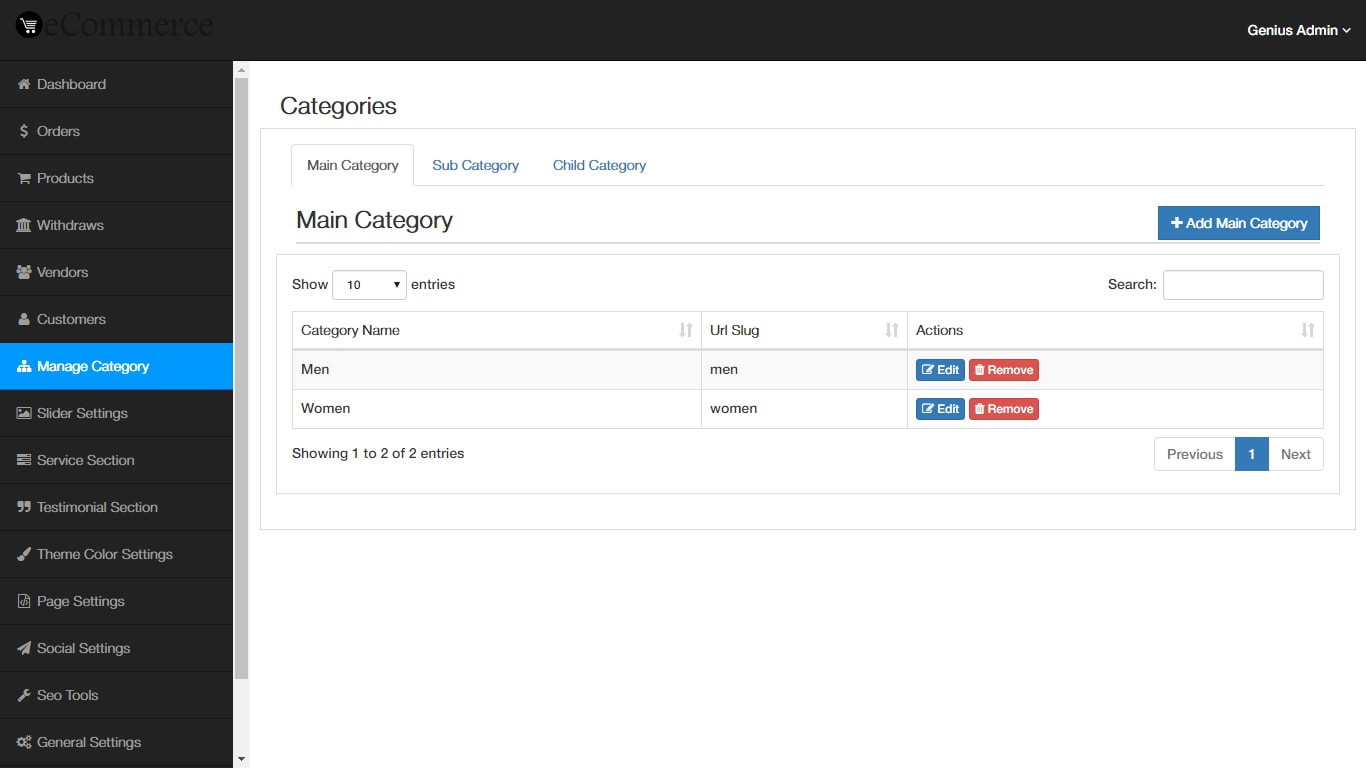This is a detailed screenshot of the Genius e-commerce admin panel interface. The layout features a two-pane design with a dark gray theme on the left side panel and top navigation bar. In the upper left-hand corner, the word "e-commerce" is barely visible in black underneath the dark gray background. The top right corner displays "Genius Admin" in white text, accompanied by a drop-down menu.

The left sidebar is a comprehensive navigation menu, highlighted in blue at "Manage Category," and includes the following options: Dashboard, Orders, Products, Withdrawals, Vendors, Customers, Manage Category, Slider Settings, Service Section, Testimonial Section, Theme Color Settings, Page Settings, Social Settings, SEO Tools, and General Settings. A vertical scrollbar next to the menu suggests additional options might be available below General Settings.

The main content area, predominantly white with black text, focuses on category management. At the top of this section, the title "Categories" is prominent. Below, a light gray box displays a hierarchy diagram where "Main Category" is selected, indicated by a gray outline surrounding it. Connected to this main category, "Subcategory" and "Child Category" are shown in blue text.

Centered below this diagram, "Main Category" is repeated in larger black text, next to a blue "Add Main Category" button with white text and a plus sign. A gray divider line crosses the entire section. Within another light gray box beneath this divider, options to display the number of entries and a search function are available. The left side offers a dropdown for showing 10 entries, while the right side has a search box labeled "Search."

The section below features a grid displaying category information. The headers are:
- Category Name (with entries "Men" and "Women")
- URL Slug (with corresponding entries "men" and "women")
- Actions (featuring blue "Edit" and red "Remove" buttons for each entry)

At the bottom, pagination details indicate "Showing 1-2 of 2." On the left is the word "Previous," while the number "1" in a blue box and "Next" are on the right, allowing navigation through potential multiple pages.

This organized, user-friendly interface supports efficient e-commerce category management through its intuitive layout and comprehensive set of options.